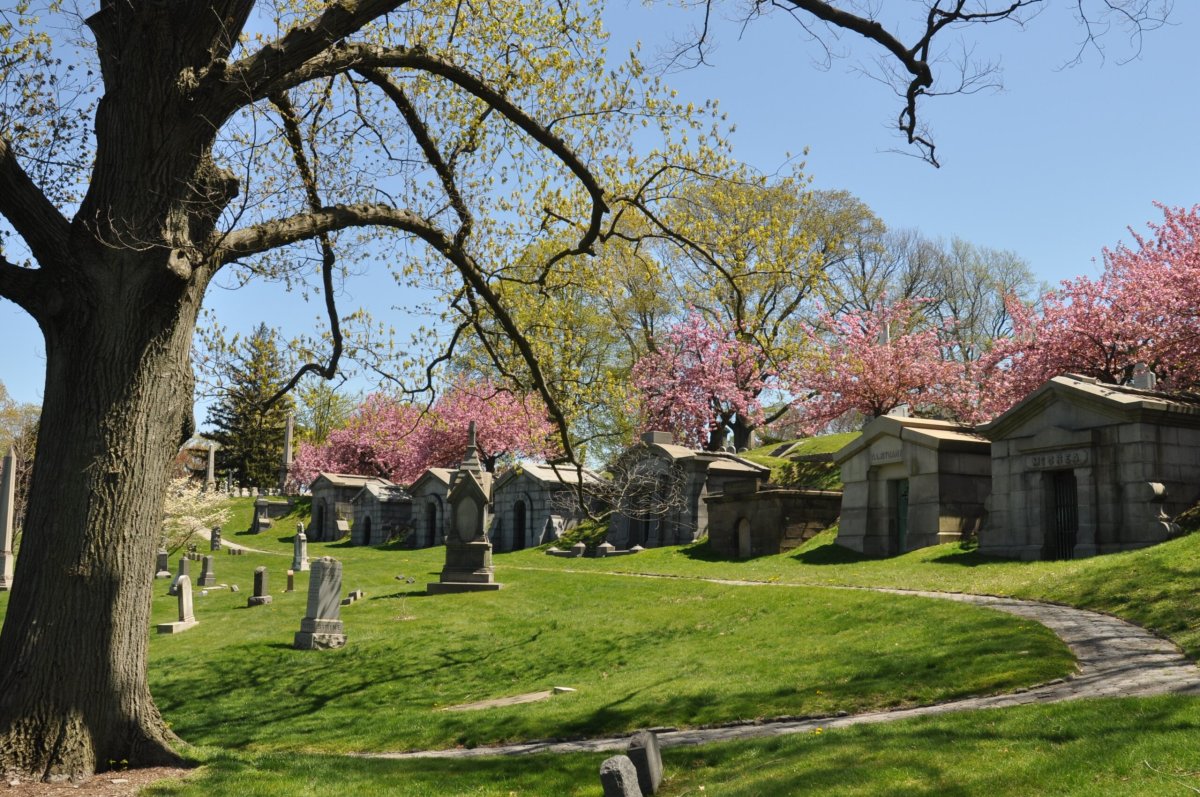This is a detailed photograph taken in an outdoor cemetery during daytime, under a clear blue sky with no visible clouds. The scene captures a slightly inclined hill from left to right. Dominating the left side of the image is a large tree with budding branches, indicating early spring. Beneath the tree are several old tombstone markers with illegible inscriptions. A brick pathway winds its way through the cemetery, meandering in front of a dozen mausoleums positioned from the right-hand side to the center of the image. These mausoleums resemble small stone buildings with gated doorways, some bearing names above their entrances. Behind the mausoleums, there are taller trees adorned with vibrant pink blossoms, adding a splash of color against the serene backdrop. Nestled among the grass and cast in the soft shadows of the trees, the cemetery's peaceful ambiance is accentuated by the bright sunlight, even though the sun itself is not visible in the sky.